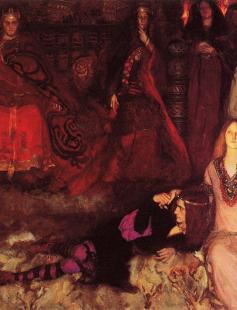The image depicts a seemingly gothic or Halloween-themed scene with an abstract and eerie atmosphere, likely intended as a portrayal from the medieval era. The focal point features two women in the foreground: one seated upright in a light pink gown with long brown hair, and another resting her head on the former's shoulder, on the floor, clad in a black dress with pink and black stockings and possibly a purple sleeve. Their surroundings are richly detailed with stark contrasts, dominated by deep reds—the background showcases a dark red wall against which another woman stands, blending into the ambiance in a long red gown, contributing to the image's unsettling tone. Additional figures with medieval attire and subtle headbands also merge with the backdrop, enhancing the haunting quality. The left side hints at a fireplace while the right is illuminated by two wall-mounted torches, with another figure cloaked in red standing there, embodying the mysterious and foreboding essence of the scene.